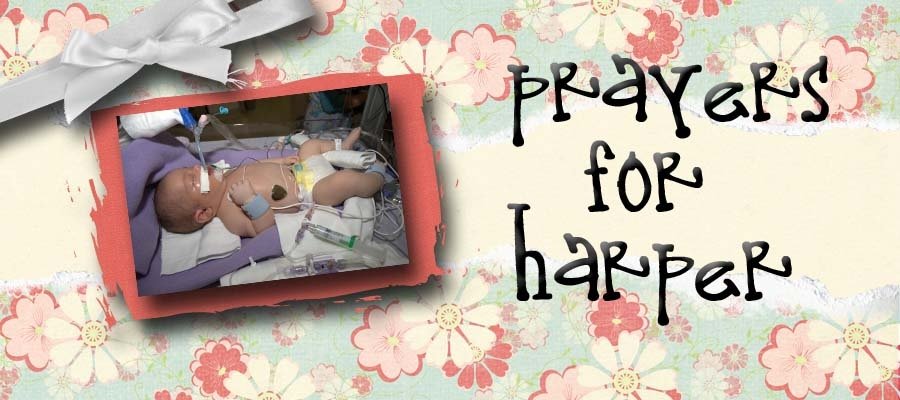The image is an intricate flyer displaying a heartfelt message amid a challenging medical situation. A newborn baby with darker skin, eyes closed, and numerous tubes connected for life support, lies in a hospital incubator, hinting at the neonatal intensive care unit (NICU) setting. The infant, with minimal hair and draped in a purple blanket, is positioned diagonally to the left. The background is adorned with a floral pattern featuring pink, white, and some blue flowers against a predominantly pink layer with underlying shadows. On the right side of the image, in distinctive black lowercase letters, the words "prayers for Harper" are inscribed, emphasizing the plea for hope and recovery. A gray ribbon in the upper left corner adds a somber, supportive touch to the overall compassionate tone of the image.